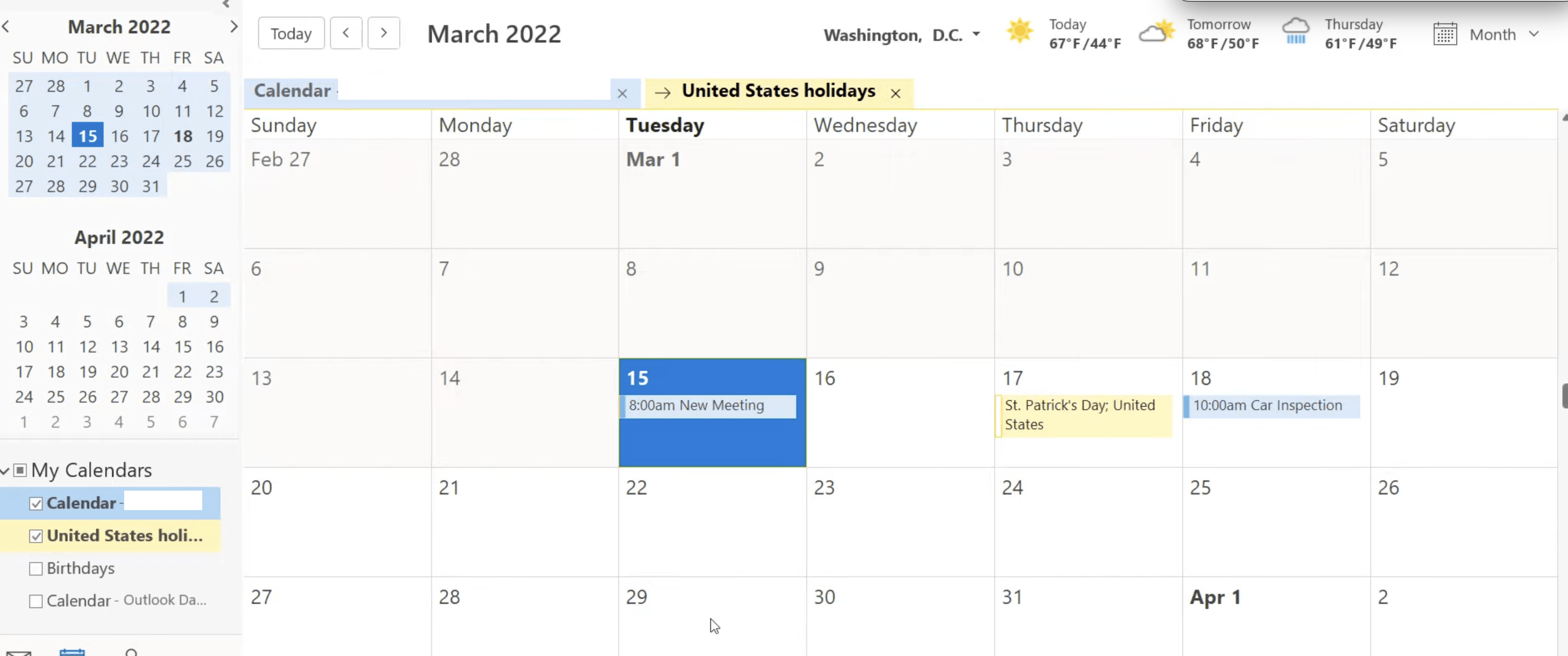The image features a detailed calendar interface primarily displaying the month of March 2022. The layout includes a weekly overview from Sunday to Saturday, with individual dates listed for the entire month. Notably, the 15th is highlighted in white text on a blue square, distinguishing it from the rest of the dates which are printed in black. The date 18th is presented in bold text for emphasis. Directly below, there is a partial view of April 2022, where the dates 1st and 2nd are highlighted with a blue background while the remaining dates are in white.

Beneath the calendar grid, there are sections labeled "My Calendars," with options such as "Calendar" in blue accompanied by a blank space, "United States Holidays" highlighted with a yellow banner, and "Birthdays and Calendar."

To the side, weather information for Washington, D.C. is displayed, showing today's date as March 22nd with a temperature forecast of 67 degrees Fahrenheit for the day and 44 degrees Fahrenheit for tomorrow.

The calendar timeline starts from Sunday, February 27th, and continues up to Friday, April 1st. Key dates include:
- March 15th: Highlighted with a blue background, noting an 8 a.m. new meeting.
- March 17th: Indicating St. Patrick's Day in the United States.
- March 18th: Featuring an event at 10 a.m. for a car inspection.